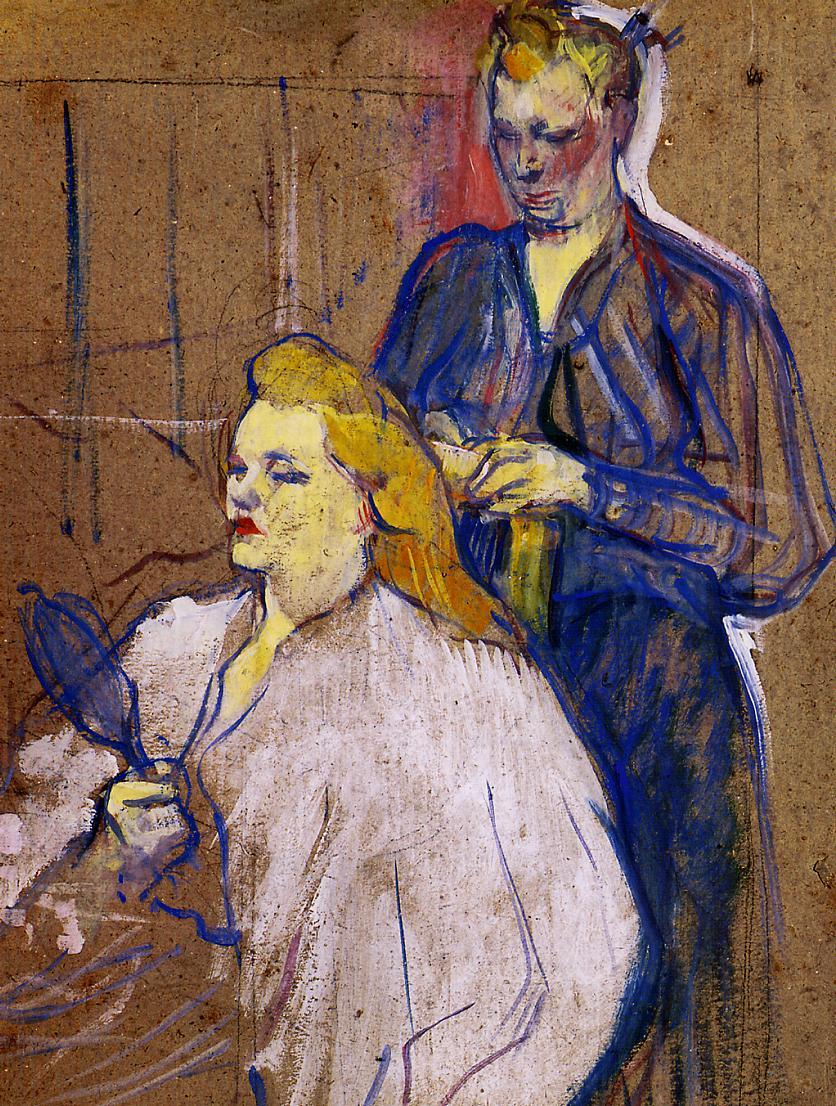In this expressive painting, two women are depicted with an impressionistic touch, characterized by broad, rough strokes and vivid colors. The scene portrays a woman on the left, seated and facing forward, immersed in her reflection as she gazes into a blue mirror held in her right hand. Her eyes are closed, and she has strikingly bright pink lips that stand out against her vibrant yellow face. She dons a voluminous white coat and her long, orange-blonde hair cascades over her shoulders.

Behind her, on the right side, stands another woman, engaged in braiding the seated woman's hair. The standing woman wears a translucent, blue-tinted dress and has a touch of yellow just below her chest, accentuating the intricacies of her attire. Her complexion blends shades of pink, amber, and yellow, crowned by brown hair interwoven with yellow and orange hues, subtly highlighted by a white silhouette around her head. 

Both women appear slightly robust and their hair is distinctive; the seated woman's hair is long and flowing, while the standing woman's hair is either shorter or styled up, possibly held by blue barrettes. The background, with its dirty brown color streaked with blue and white and dotted with black speckles, forms a textured yet indistinct backdrop, bringing the focus sharply onto the intimate interaction between the two women.